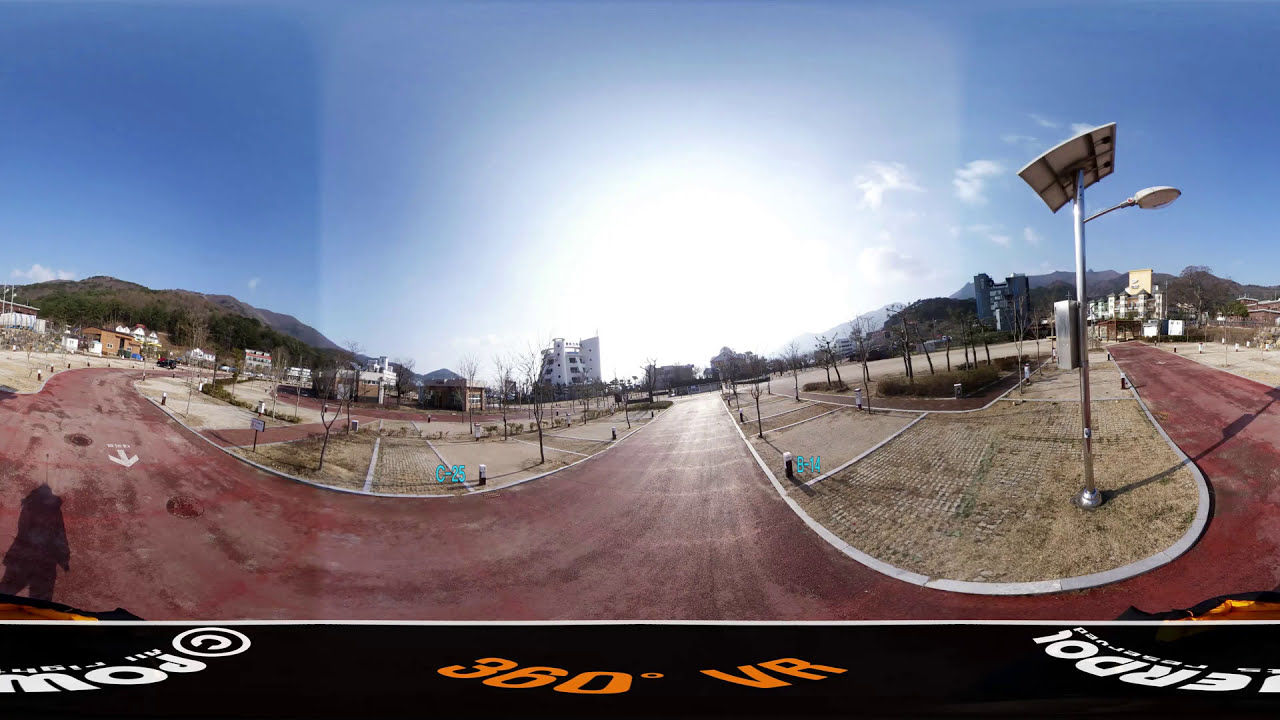The image is a panoramic shot of a newly made, curved red road that resembles a W with smooth, rounded ends. This road lacks distinct lane markings and street lamps are present along its stretch, giving it an almost racetrack-like appearance. The surrounding area includes patches of grass and newly planted, leafless trees, suggesting it might be wintertime. In the background, there are several buildings, including a tall white five-story building and a black twelve-story building. Scattered smaller buildings appear closer to the road, behind which a brown mountain with green tree-covered lower slopes is visible. The vast expanse of blue sky takes up most of the picture, emphasizing the emptiness, as there are no cars or people present. A text at the bottom indicates the image was taken with a 360 degrees VR perspective.